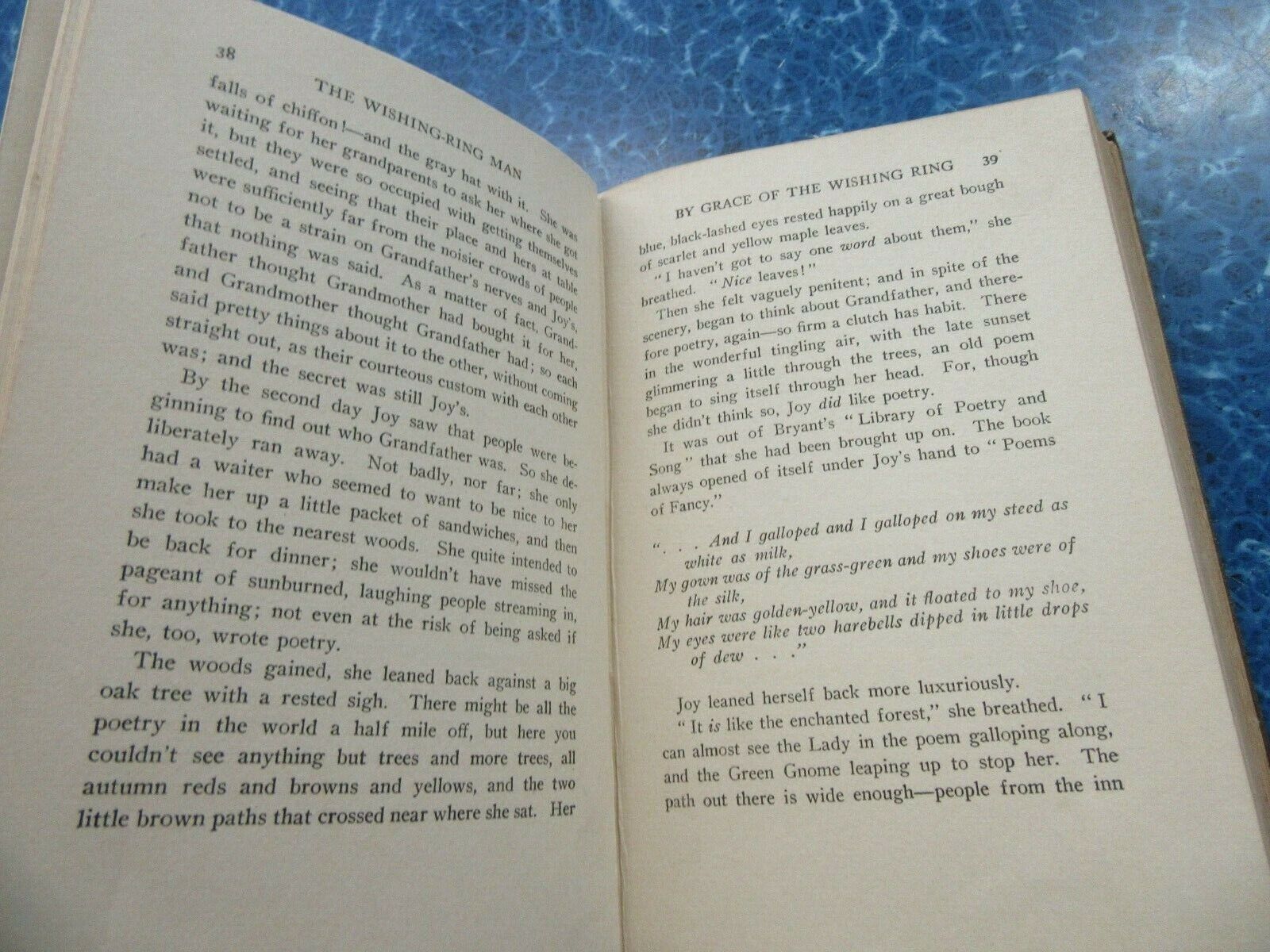The image depicts an open book titled "The Wishing Ring Man" by Grace of the Wishing Ring, resting on a blue and white marbled or crackle-patterned countertop. The book is open to pages 38 and 39, where the text begins with "Falls of chiffon and the gray hat with it." The narrative describes a character named Joy, who is waiting for her grandparents to inquire about something she has, but they are preoccupied with ensuring their seating arrangements are away from the noisier crowds to avoid straining Grandfather's nerves. Both grandparents mistakenly believe the other has acquired it for Joy, leading to a polite exchange with each other while the secret remains with Joy. The passage continues, detailing Joy's brief adventure into the woods to avoid being recognized, her contemplation under a grand oak tree, and her musings on poetry, specifically from Bryant's library of poetry and song. The detailed autumn setting and Joy's literary reflections convey a deep sense of peace and appreciation for nature's beauty.